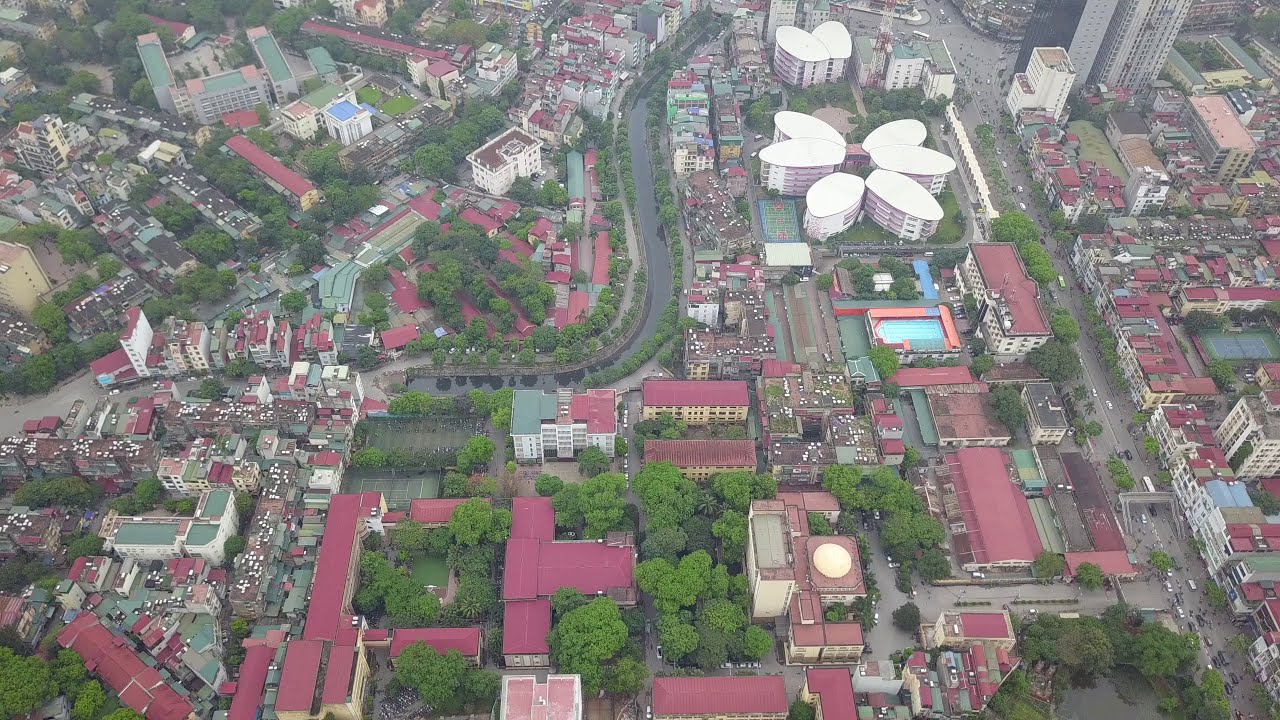This aerial image captures a densely packed town or city with predominantly low-level, red-roofed buildings, situated amidst lush, puffy deciduous trees. Dominating the lower half of the rectangular frame, these buildings line a network of streets bustling with cars. Central to the scene is a winding canal or river that gracefully curves around the city, adding a serene element to the urban landscape. Notably, in the middle of the image, a distinctive cluster of white-roofed buildings forms a striking flower-like pattern, possibly representing condos or a hotel, each equipped with balconies overlooking nearby tennis courts or a swimming pool. In the upper right corner, the view extends towards a truncated skyscraper standing at the end of a long, narrow street. The presence of broad white avenues, the absence of visible people, and the sunlight illuminating the scene suggest that this high-altitude shot, possibly taken by a drone, captures the town in the full light of day. The overall composition highlights the harmonious blend of urban structures and natural greenery.